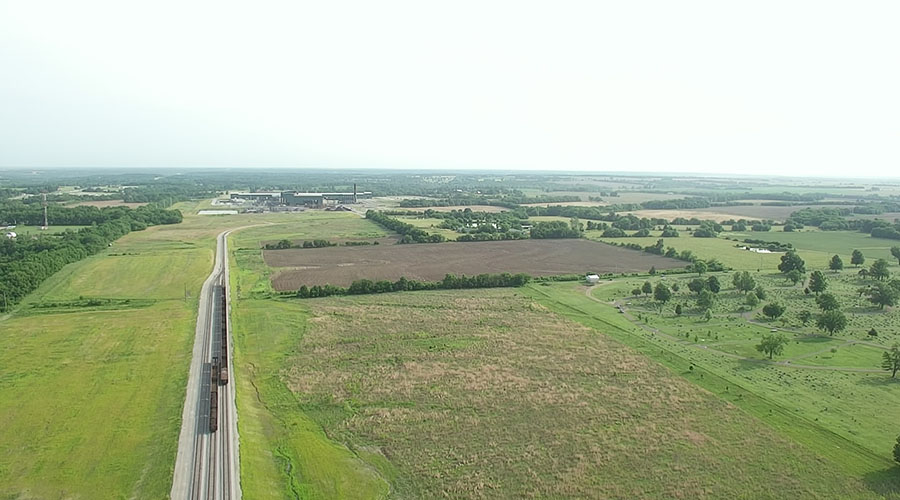The image is a panoramic, aerial photograph taken during the daytime, capturing a vast, flat landscape under an overcast blue sky. The shot encompasses several green fields extending across the frame, with a prominent set of railroad tracks in the lower foreground. These tracks, three in number, converge into one track that disappears into the distance. Two trains are visible, with one traveling on the center track and the other on the rightmost track.

Adjacent to the train tracks on either side, expansive fields stretch out, some of which appear to be cultivated. A noteworthy rectangular plot of land, situated near the top center of the image, has been cleared of grass and tilled, likely for planting. This dirt field contrasts sharply with the surrounding greenery. Scattered sporadically across the landscape, groves of trees and individual trees punctuate the fields, adding variety to the scene.

Additional details include patchy grass areas and a reddish-brown dirt field in the foreground. In the distance, buildings and other structures are faintly visible, suggesting that the railroad tracks may lead to a station or inhabited area. The photograph, captured in color, represents the scene with a high degree of realism typical of drone photography.